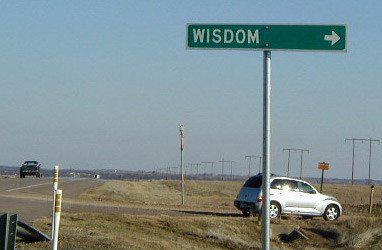A photograph taken in a very flat, open area depicts a silver metal pole in the foreground, which supports a green rectangular sign that reads "Wisdom," with a white arrow pointing to the right. The landscape is marked by mostly brown and white grassy vegetation, sand, and several electrical poles that stretch towards the horizon on the right-hand side. On a horizontal road, a silver hatchback SUV is traveling to the right. A dark-colored pickup truck is seen driving away on a vertical road to the left. Additionally, there's a stop sign across from the "Wisdom" sign, viewed from a side angle. The scene captures the vast, desolate nature of the area juxtaposed with the sparse traffic and minimal signage.